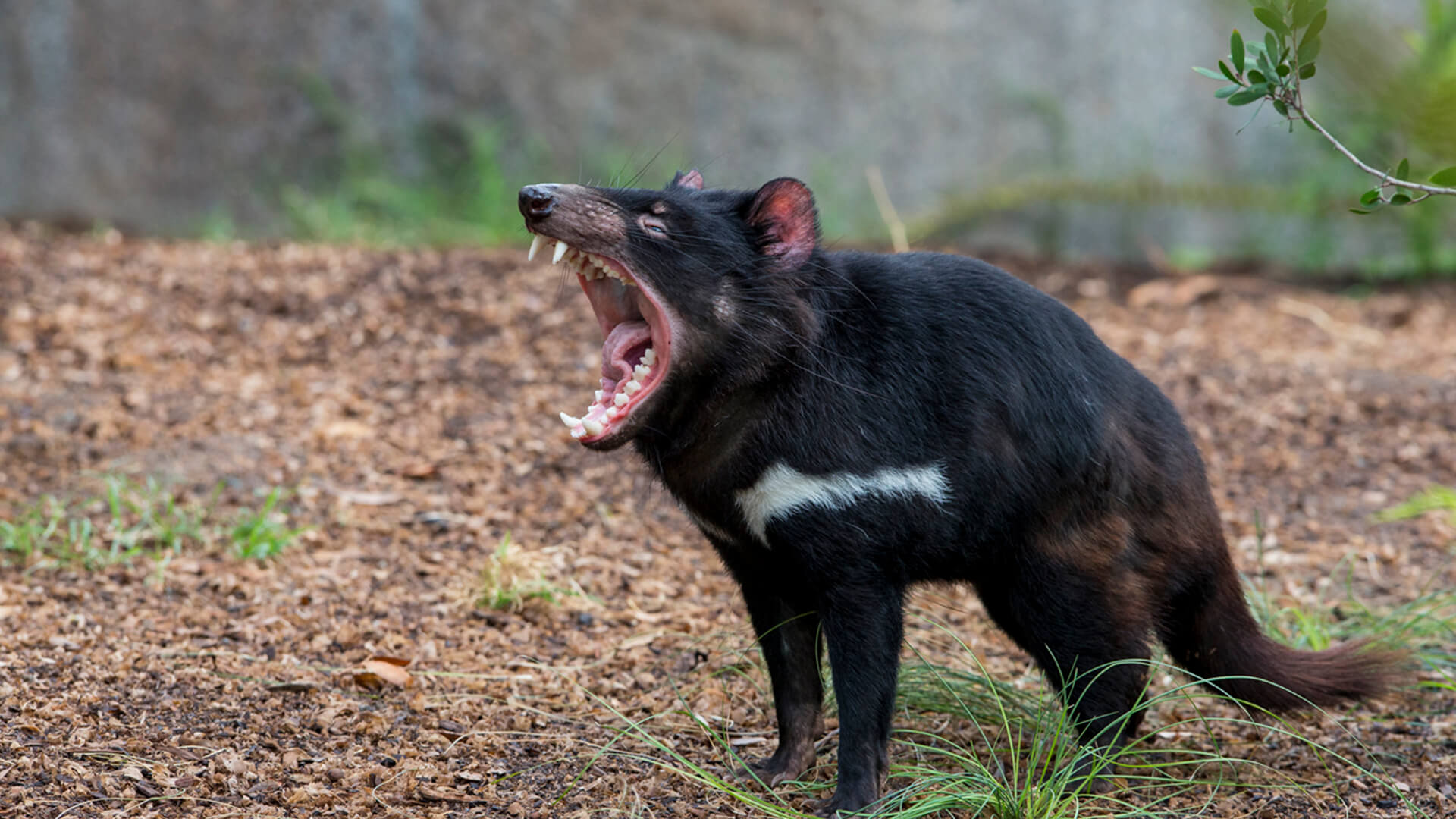This photograph captures a black Tasmanian devil in its natural habitat, presumably in Australia, based on its appearance and features. The animal is small and low to the ground with a bushy brown tail and a body that includes black fur accented by a white patch on its upper left shoulder extending towards its mid-back. The creature, which has a face similar to a rat but with a larger body and longer legs, is shown mid-yawn, exposing its sharp teeth, a slightly bent tongue, and revealing the top and bottom fangs distinctly. The Tasmanian devil is situated on a mostly flat, dry, brown ground scattered with wood chips and patchy grass, surrounded by sparse shrubbery. In the background, a gray sky looms above the bases of several large tree trunks and patches of green grass interspersed with dry leaves, portraying a rugged, outdoor environment.